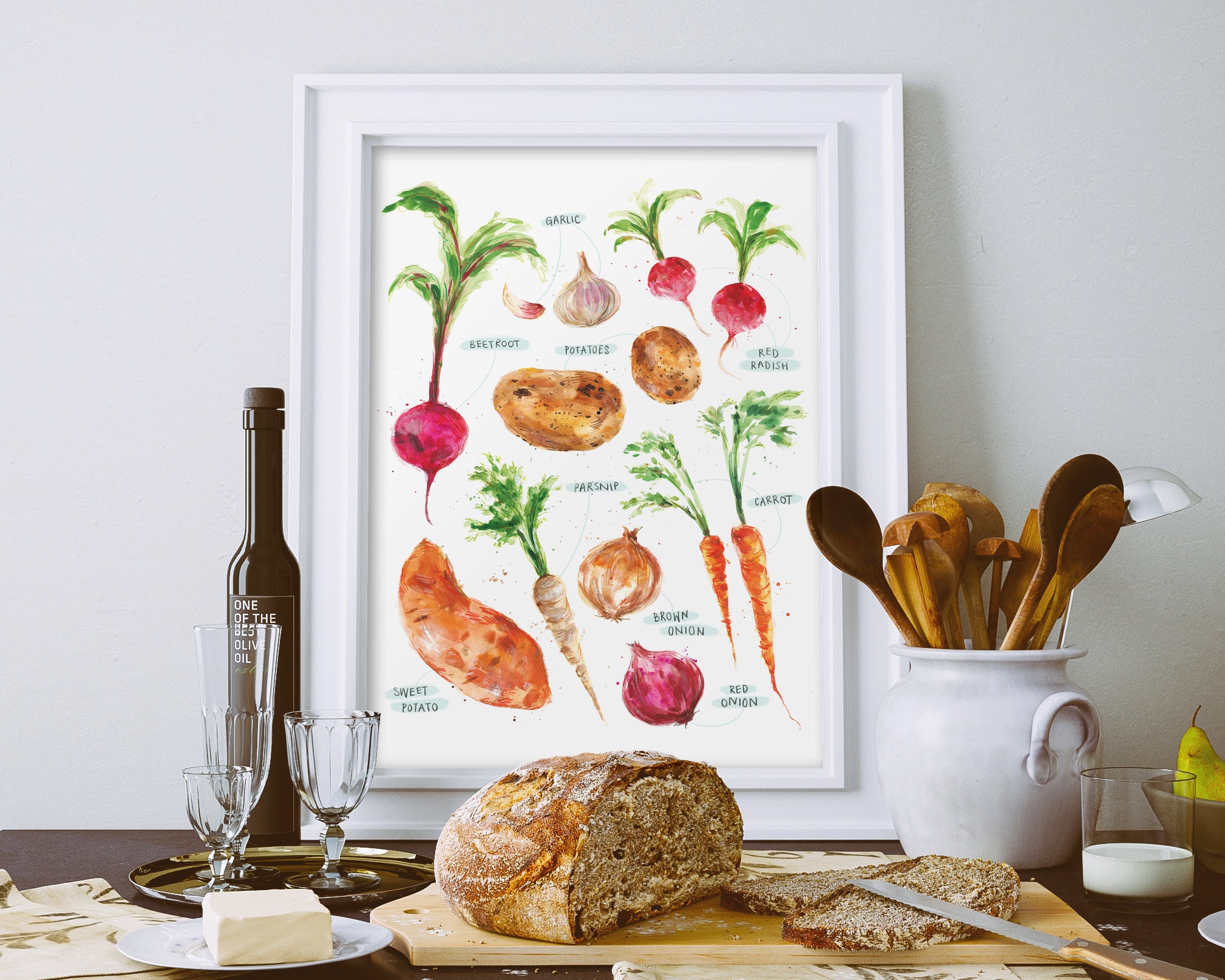The image depicts a cozy kitchen or dining room with a light gray wall in the background. In front of the wall stands a dark brown table, which prominently features a light brown cutting board that holds a rustic, artisanal rye loaf of bread. Two slices are positioned in front of the loaf, and a long bread knife with a silver blade and a tan handle rests on top of the slices.

To the left of the cutting board is a small white plate containing a stick of butter. A black, round tray behind the plate holds three empty glasses of various sizes and a tall, slender bottle of olive oil labeled "One of the best olive oil." On the right side of the table, beside the cutting board, is a glass of milk filled just at the bottom, and a round, white vase containing multiple wooden kitchen utensils like spoons and juicers.

Against the wall hangs a white-framed print illustrating an array of vegetables, including garlic, beetroot, potatoes, red radish, carrots, a brown onion, a red onion, and a sweet potato. The overall scene evokes a warm, rustic atmosphere, blending various elements of utility and decor.